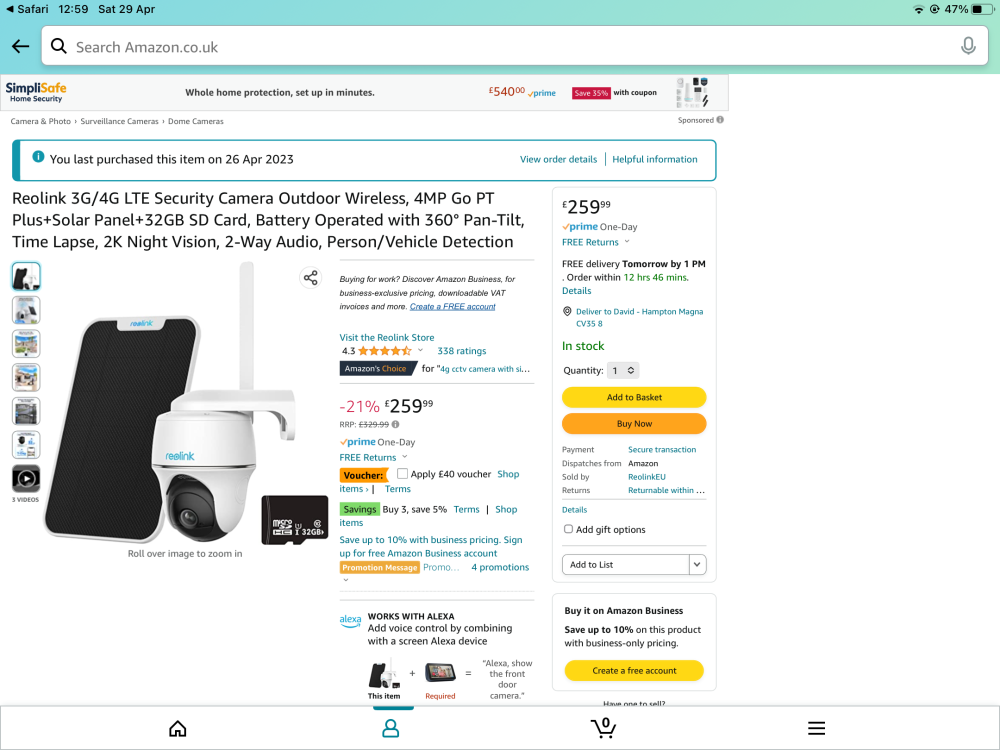Detailed Description of the Amazon UK Product Page:

The image depicts an Amazon UK search result page displayed on a Safari web browser. The search conducted is for a security camera, specifically a "SimpliSafe Home Security" system. The screenshot was taken at 12:59 PM on Saturday, April 29th.

On the left side of the browser, there's a black arrow pointing to the search bar which reads, "search amazon.co.uk." The product featured is a Rulink 3G/4G LTE Wireless Security Camera. Key features of the camera include 360-degree pan/tilt functionality, a solar panel for power, night vision capabilities, two-way audio, and person/vehicle detection.

The camera is currently priced at £259, reflecting a 21% discount. There's a promotional offer where customers can apply a £40 voucher to further reduce the price. Additional savings include a 5% discount when purchasing three cameras. For Amazon Prime members, the product is eligible for one-day delivery, with an estimated arrival by 1 PM the next day if ordered within the next 12 hours and 46 minutes, as indicated on the screenshot.

The product is noted to be in stock and ready for delivery to the address "David Hampton, Magna, CV 358." Only one camera has been ordered in the screenshot. The Rulink camera is white and compatible with Alexa for smart home integration. It includes an option to insert a memory disc for data storage. The product page also features various images demonstrating potential installation locations and usage scenarios.